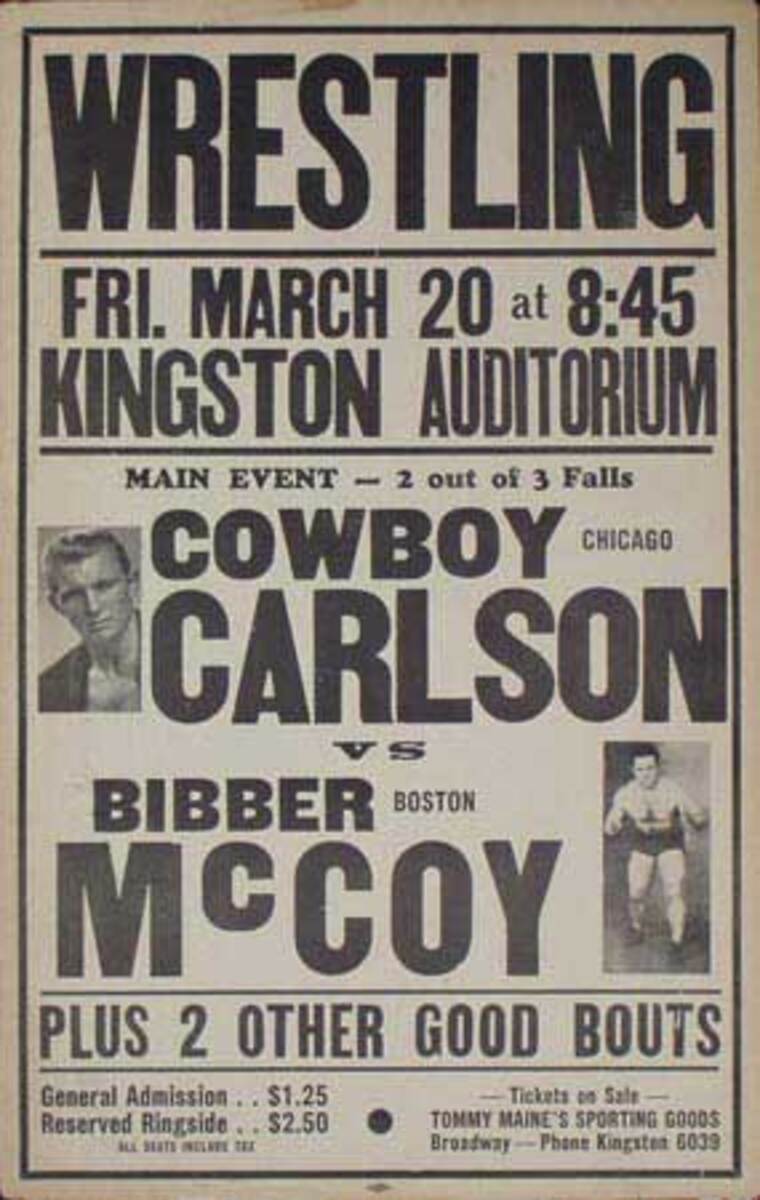Black and white advertisement that appears to be an old flyer or newspaper clipping for a wrestling event. The top of the ad features the bold text "This is Wrestling" with a black border above and below. It announces the event on Friday, March 20th at 8:45 PM at Kingston Auditorium. The main event is a two out of three falls match between Cowboy Carlson, depicted in a headshot as a blonde man with a model-like appearance, and Bibber McCoy, shown in a full-body shot as a muscular man wearing shorts and in a fighting stance. The ad also mentions two other good bouts. Ticket prices are listed at the bottom of the ad: general admission for $1.25 and reserved ringside for $2.50. Tickets are available at Tommy Maine Sporting Goods on Broadway, with the contact phone number Kingston Black 5039.